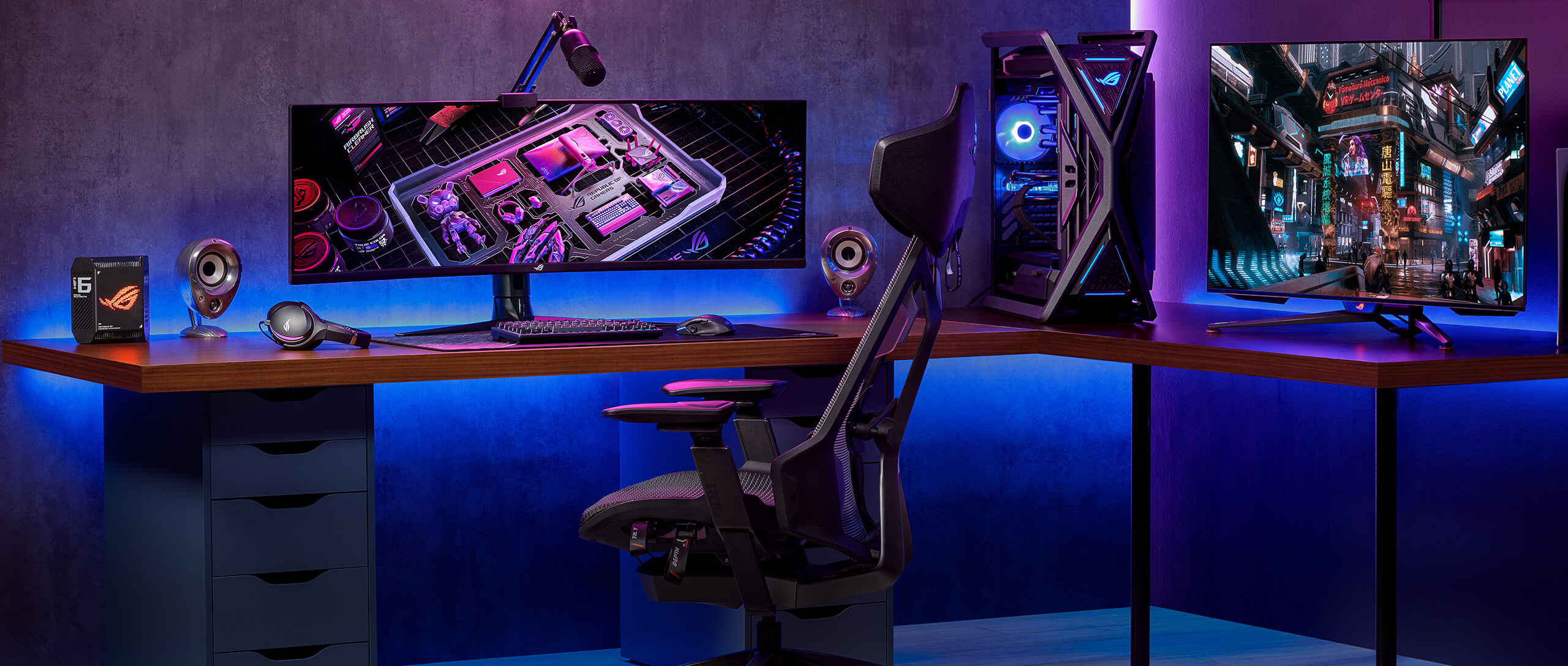In this detailed photograph of a high-end gaming workspace, an impressive L-shaped wooden desk with thin wood top spans the scene. On the left side of the desk sits a set of blue drawers, while black supports or posts hold up the worktop on the right. The centerpiece is a sleek black gaming chair positioned in front of a sophisticated, dynamic setup, suggesting the space belongs to a dedicated gamer or streamer. 

To the left of the desk, a massive curved ultra-wide monitor is flanked by a keyboard, mouse, and a microphone mounted on its top, hinting at potential streaming or podcasting activities. Nearby speakers indicate an immersive audio experience. The right side of the desk features a standard 16x9 monitor displaying a game, accompanied by another keyboard and mouse. Between these monitors, strategically placed in the corner of the desk, resides a high-performance desktop PC illuminated with blue LED lights, possibly signifying advanced components like liquid cooling.

Additional key accessories such as a headset and a webcam sit near the curved monitor, completing the professional setup. The ambiance of the room is enhanced by a blue and purple lighting effect, casting a futuristic, almost digital artist-rendered quality to the photograph, which emphasizes the modern and expensive aesthetic of the workspace.